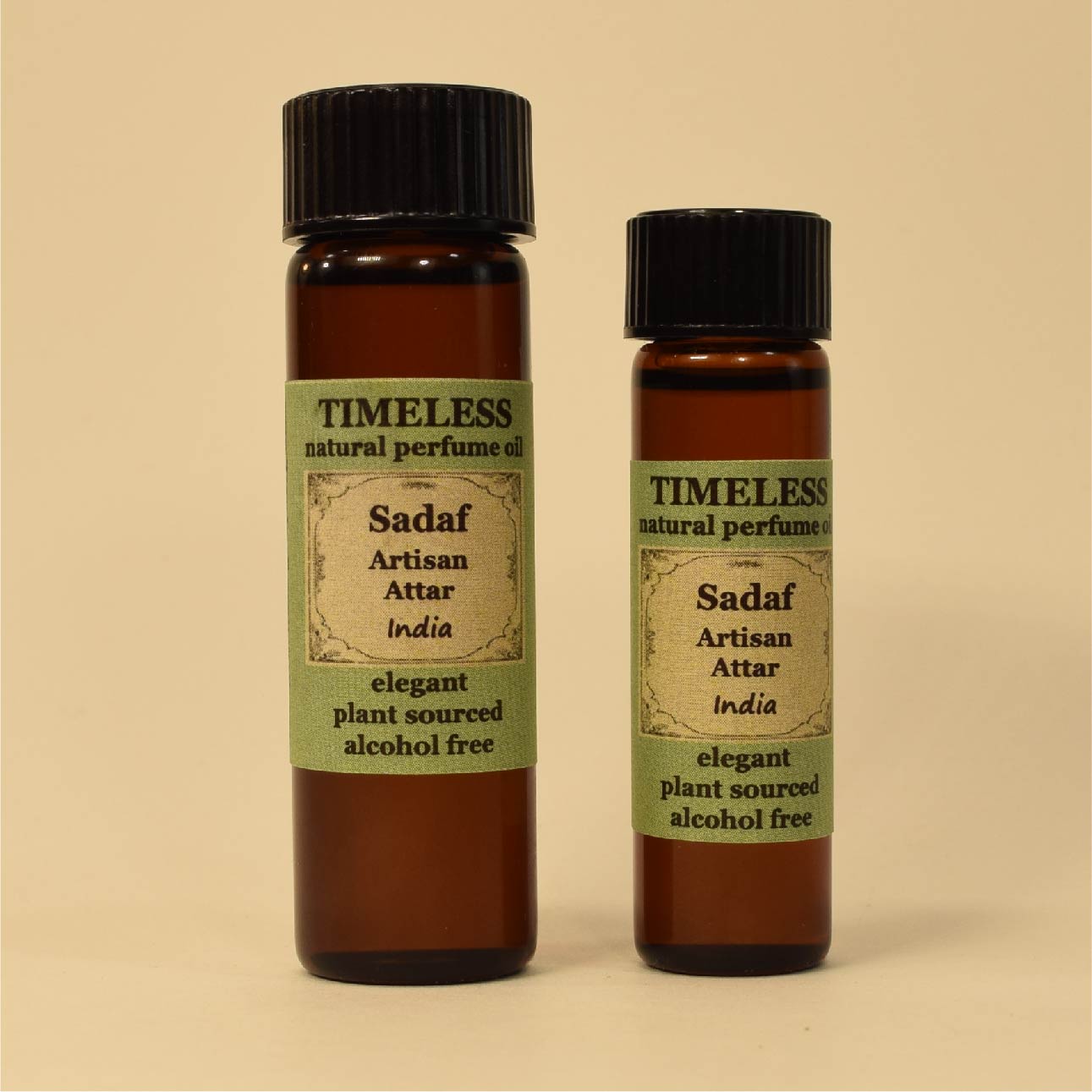This square photograph, measuring approximately 5 to 6 inches in both height and width, features an indoor scene with a seamless brownish-peach background that lacks distinguishing lines to separate the ground from the back. Central to the image are two amber cylindrical vials, each capped with black, easily twistable plastic tops. The taller vial on the left stands around 4 inches high and an inch wide, while the smaller vial on the right measures roughly 3 inches in height and three-quarters of an inch in width. Both vials contain a visible liquid and are adorned with green labels. The top of these labels bears the inscription “Timeless Natural Perfume Oil” in black print, while the bottom reads “Elegant Plant Sourced, Alcohol Free.” A light brown square with black text in the center of the label states “SADAF Artisan Attar India.” The label details and color coordination harmonize with the tan-brownish hues of the background, creating a visually coherent presentation.